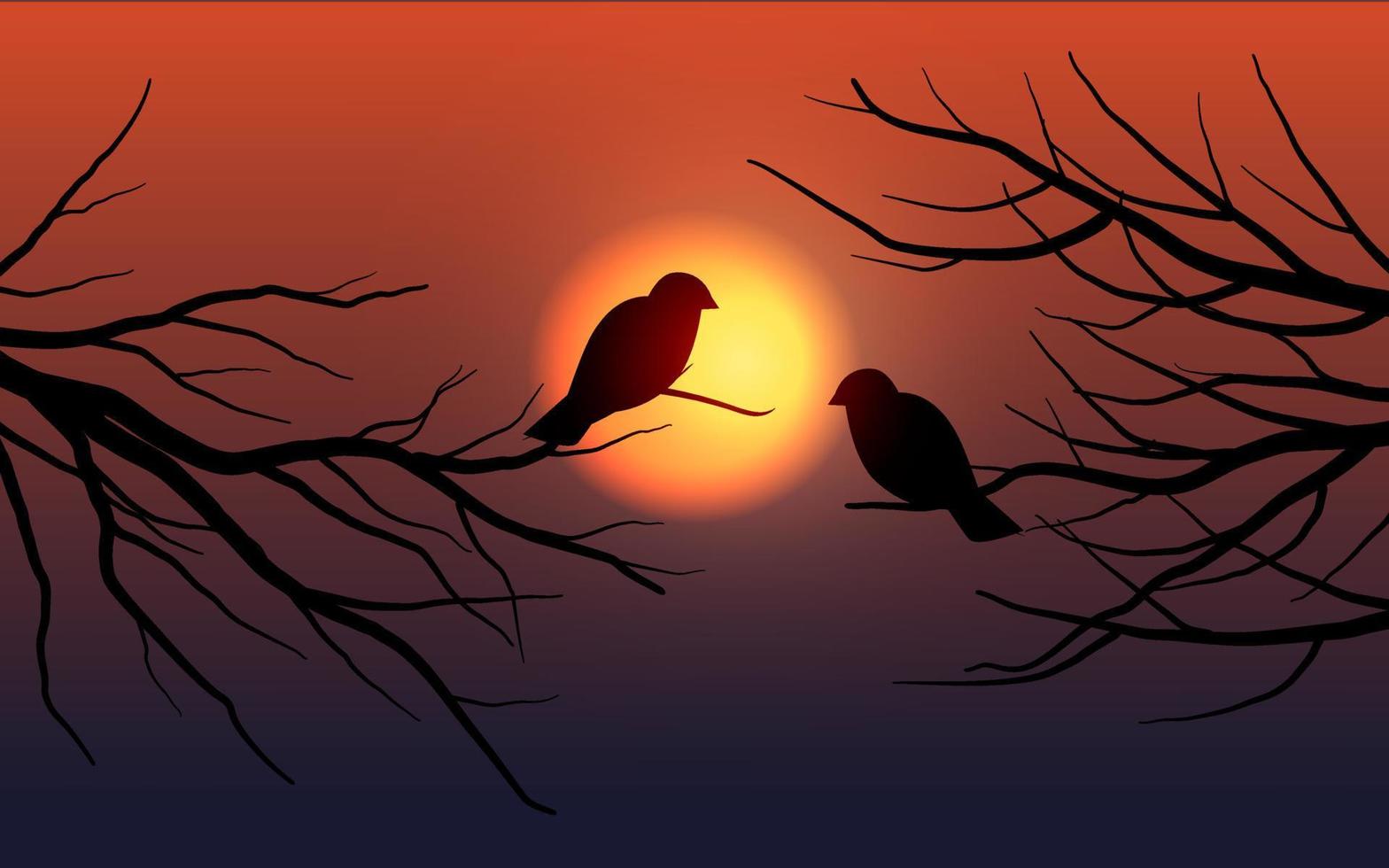Against the vibrant hues of a setting sun, which transitions from a central yellow to deep orange and ultimately to a dusk-like azure, two silhouetted birds are perched on bare tree branches. These birds, perhaps sparrows or doves, are positioned on opposite sides of the image. The left bird sits starkly against the glowing sun, enhancing its dark outline, while the right bird appears to be mid-flight or just landing. The scene captures a tranquil moment just before nightfall, with the orange and yellow gradient of the sky casting a serene backdrop, devoid of any text, but rich in natural beauty and atmosphere.